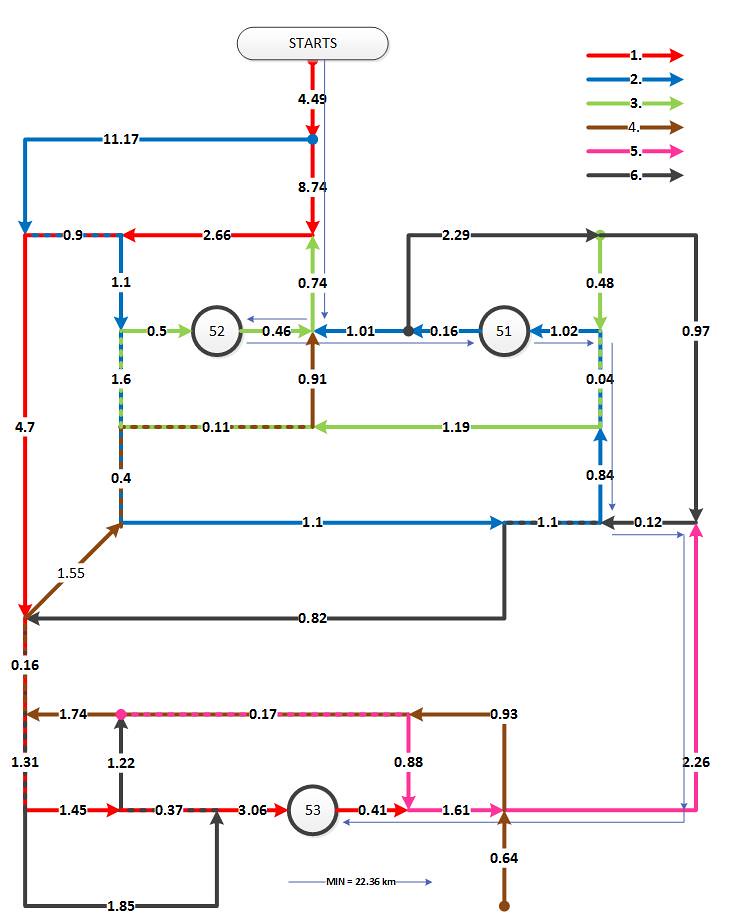The image depicts a detailed flow chart set against a white background, featuring a complex network of lines, arrows, and numerical values, all rendered in a variety of colors including red, blue, light green, brown, pink, and black. At the top center, a circular node labeled "Start" initiates the chart.

From this starting point, a red arrow directs the viewer rightward, leading into a blue line with a length of 4.49 units. This blue line continues left for an additional 11.17 units before descending 8.74 units. It then extends right for another 0.9 units. Subsequently, a red line takes over, moving from left to right for 2.66 units. Directly below, a green line drops 0.74 units.

The chart comprises approximately 20 to 30 such lines of varying lengths, each annotated with numerical values that likely denote specific measurements between connected points. Taken as a whole, the flow chart appears to map out intricate pathways and their corresponding dimensions, spanning an estimated grid area equivalent to about 9.7 units vertically and roughly 7 units horizontally.

Overall, the chart serves as a visual representation of a complex process or system, with each line and arrow meticulously illustrating the distances and connections between successive points.